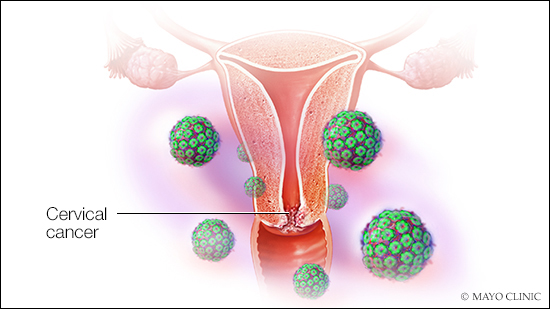The image is a detailed medical diagram of the female reproductive system, specifically highlighting the cervix, and is likely sourced from a medical textbook. Positioned on a white background and bordered by a black outline, the diagram prominently features the pink cervix, which is outlined in white. The cervix is positioned centrally within the illustration, with the fallopian tubes extending from each side. At the base of the cervix, where it narrows into the vagina, there is a black line pointing to this area, labeled "Cervical Cancer" in black lettering on the left. Surrounding the cervix, numerous balls are depicted; each has a green exterior with a red center, representing cervical cancer cells. These cells vary in size and are scattered throughout the area. The bottom right corner of the image includes a copyright attribution in black, stating "Mayo Clinic," confirming the source of the diagram.